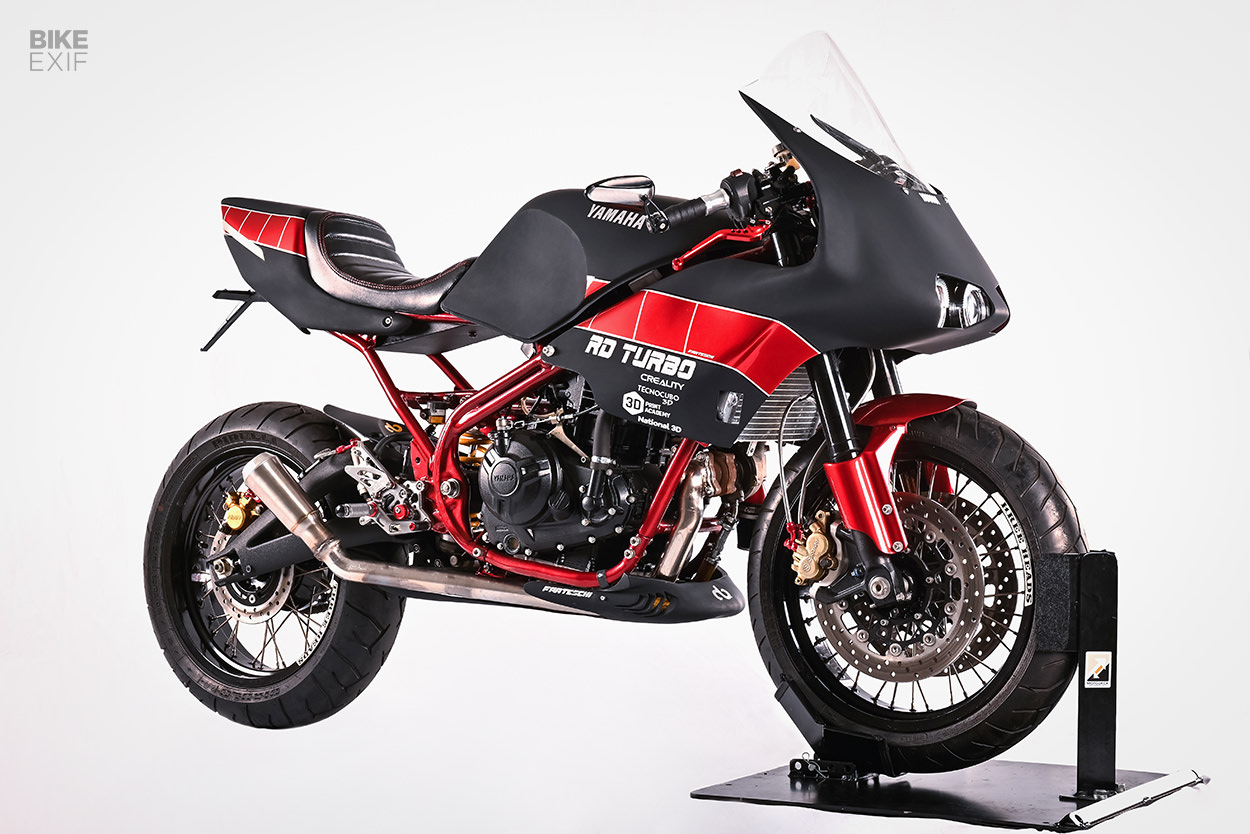This detailed photograph showcases a Yamaha RD Turbo motorcycle, elegantly suspended on a black floor stand that securely braces the front wheel. The motorcycle, facing to the right, is primarily black with striking red accents that highlight its sleek design. The engine is encased in red metal, complemented by smooth black plastic grilles and a clear visor screen for the rider. The tires are black with intricate golden elements and silver spokes, adding to the bike's sophisticated appearance. The image is photorealistic, capturing the fine details of the motorcycle's construction, and is set against a pristine white background, emphasizing its features. The hatchback scoop seat and distinct red squares and rectangles bordered in white further accentuate the bike's unique design. The black stand ensures the motorcycle is perfectly stable and appears to be on display, highlighting its aesthetic and functional elements.